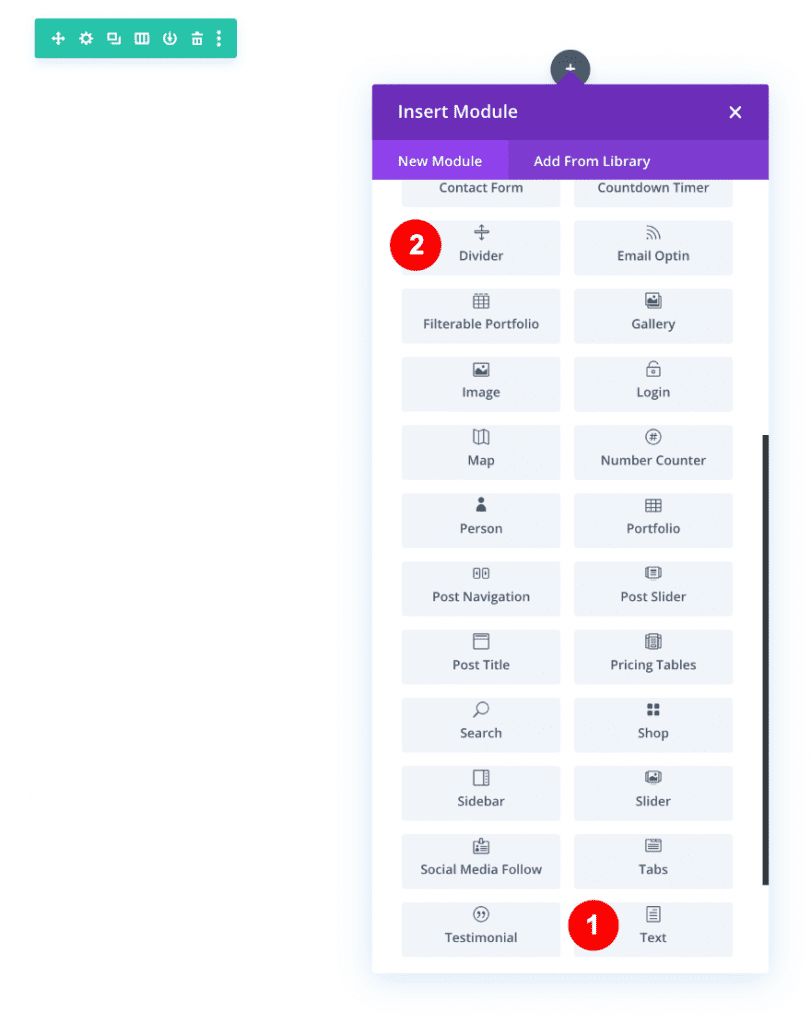The screenshot showcases an interface from an Android mobile device, featuring a purple header bar at the top labeled "Insert Module" accompanied by a white 'X' for closing the module on the right side of the header. Directly below this header, there are two purple tabs: "New Module" and "Add from Library." The "New Module" tab is highlighted in a slightly lighter shade of purple, indicating it is currently selected.

Beneath these tabs, the screen is divided into two columns consisting of approximately 24 clickable icons for adding new modules. These icons are organized in a grid and feature various functionalities. Two of these icons are distinctly labeled with red circles containing white numerals for easy identification. The first labeled icon, marked with the number 1, is found at the bottom right corner and is identified as "Text," symbolized by an icon of a piece of paper with writing. The second labeled icon, marked with the number 2, is located at the top left corner of the visible section and features an icon of a plus sign labeled "Divider."